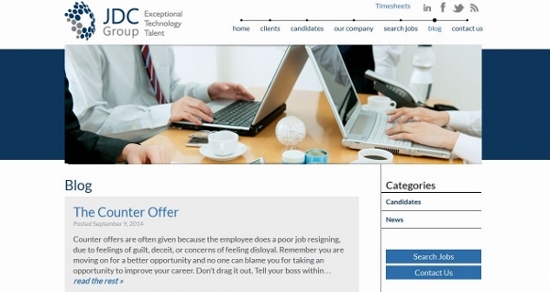This detailed caption describes an image from JDC Group, highlighting various visual elements within the image and its context on a webpage.

---

The image is from the JDC Group website and prominently features their tagline, "Exceptional Technology Talent." JDC Group's logo, a cluster of dots forming a circle, is visible. The website’s navigation bar includes options: Home, Clients, Candidates, Our Company, Search Jobs, and Contact Us. There are also links for Timesheets, Facebook, Twitter, and LinkedIn. The main photograph shows two people sitting opposite each other at a wooden table, both working on laptops. One man, who is wearing a tie, is visible, while only the hands of the other individual can be seen, suggesting he might be another man. An additional arm, possibly belonging to a person wearing a black jacket (potentially a woman), is also visible. Coffee cups are scattered on the table, and it looks like there may be another person sitting at the table's end. The photograph is framed by blue bars on the left and right. Below the image, there is a blog section titled "The Counter Offer," discussing the topic of counter offers in employment, touching on issues like guilt, deceit, and disloyalty when resigning from a job. This section advises employees to move on for better opportunities and to inform their boss promptly. On the other side, there are category links in blue, including Candidates, News, Search Jobs, and Contact Us.